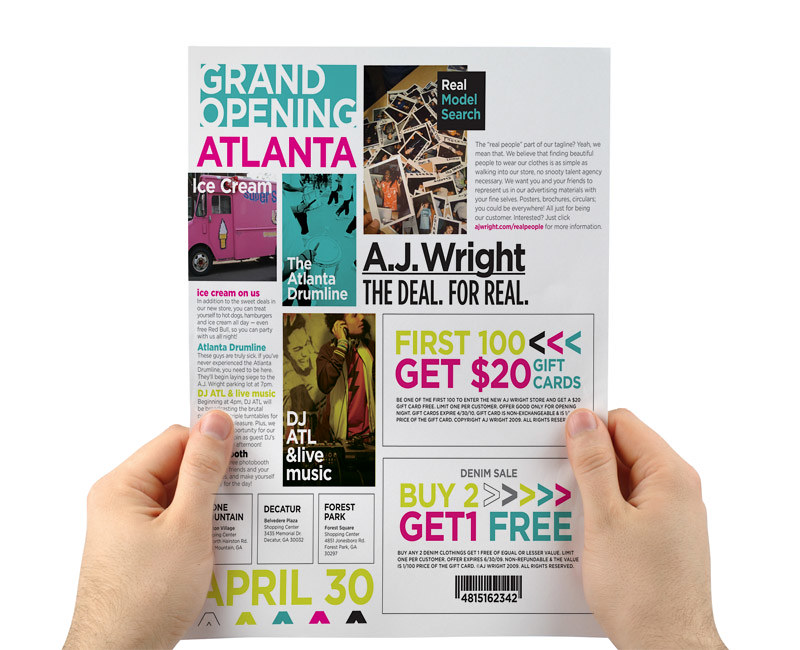The image features a pair of hands, likely those of a white man, holding a white piece of paper from the wrist up. This advertisement has a vibrant design with colorful text in shades of teal, pink, yellow, and black. At the top left, it announces "Grand Opening Atlanta" in a colorful, bold font. Below that, in large letters, it promotes "Ice Cream on Us," followed by the Atlanta drum line’s participation, "DJ ATL," and live music, all set against a mix of blue and pink backgrounds. 

On the upper right, the ad highlights a "Real Model Search" for AJ Wright with images of Polaroids scattered around. Further down, the paper includes enticing coupons: "First 100 get $20 gift cards" in a yellow section, and a "Denim Sale - Buy Two, Get One Free" offer with a barcode next to it. The text "April 30" is prominently placed at the bottom, suggesting the date of the event. The entire composition appears to be part of a magazine, held in a professional photo shoot setting with a white backdrop, emphasizing the neat, promotional layout of the flyer.